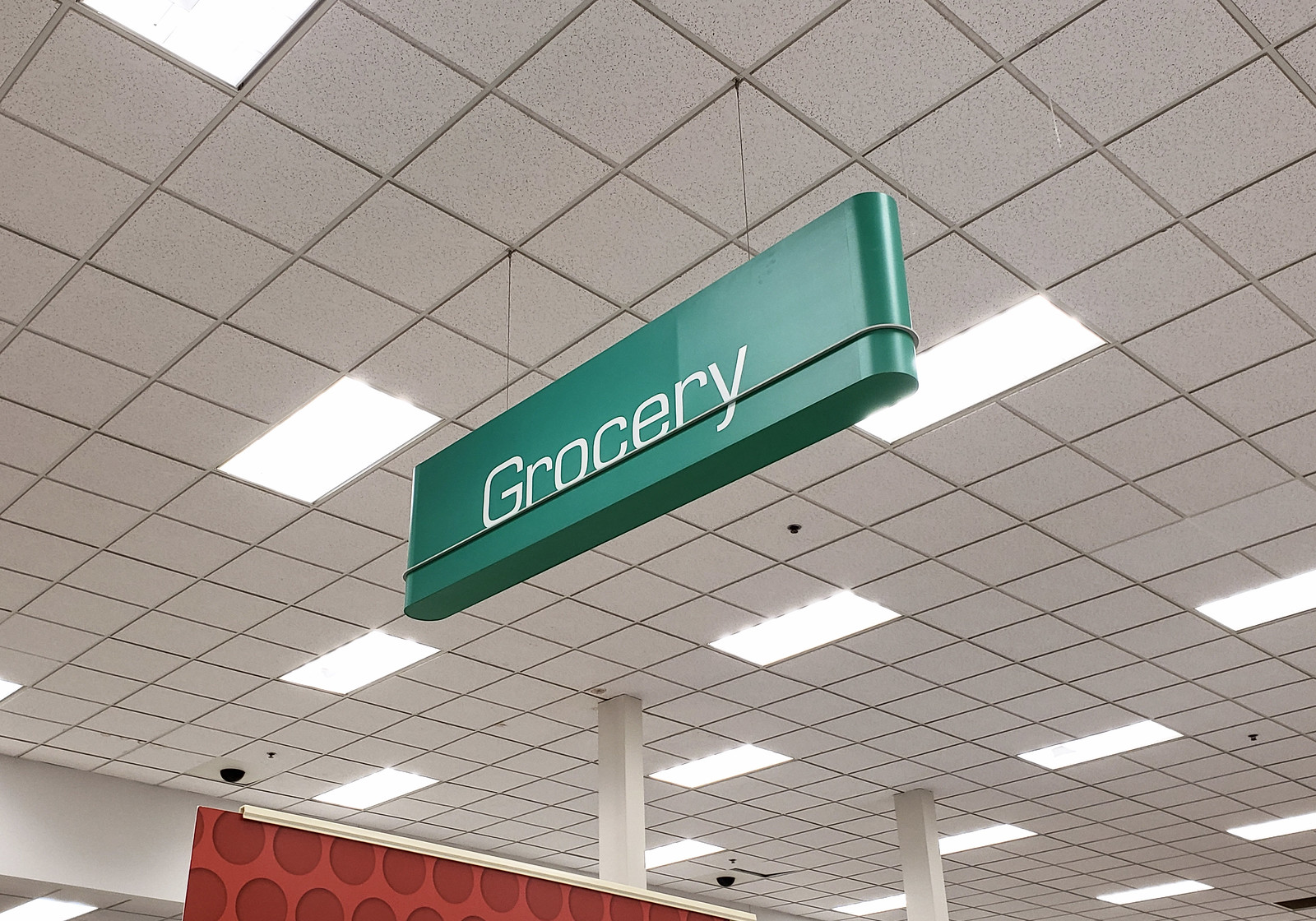The image captures the interior of a building, likely a grocery store, as suggested by a prominent green sign hanging from the ceiling with the word "Grocery" written in white font. The sign is suspended by two strings or lines and features an additional horizontal line underneath the word "Grocery." The ceiling is composed of a grid of white square tiles, interspersed with rectangular white lights that span the length of two tiles each. In the background, two white columns descend from the ceiling, and a red structure adorned with darker red circles is also visible.